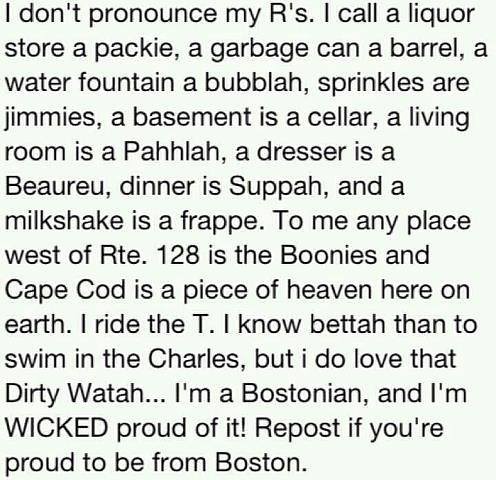The image features a light green background with prominent black text that humorously captures the essence of a Bostonian's local dialect and cultural quirks. It reads: "I don't pronounce my R's. I call a liquor store a packy, a garbage can a barrel, a water fountain a bubbla, and sprinkles jimmies. A basement is a cellar, a living room is a parlor, a dresser is a bureau, dinner is supper, and a milkshake is a frappe. To me, any place west of Route 128 is the boonies, and Cape Cod is a piece of heaven here on Earth. I ride the T. I know better than to swim in the Charles, but I do love that dirty water. I'm a Bostonian, and I'm wicked proud of it. Repost if you're proud to be from Boston." The image encapsulates regional vernacular and pride, resonating deeply with Boston locals.